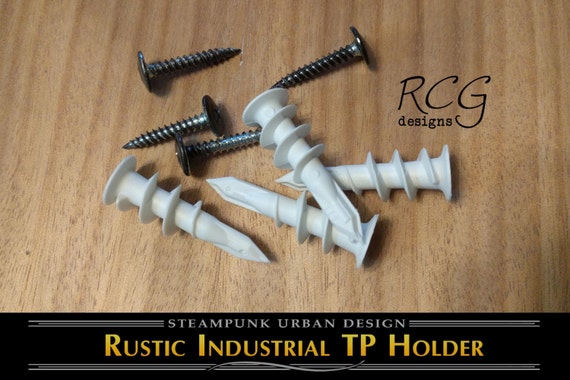The image is an advertisement poster featuring a display of screws on a brown wooden surface. There are eight screws in total: four small metallic screws in black and silver, and four larger white screws that appear to be plastic. The screws are positioned randomly on the surface. To the right side of the image, there is a watermark in black letters that reads "RCG designs." At the bottom of the image, a black horizontal strip displays the text "Steampunk Urban Design" in black letters, followed by "Rustic Industrial TP Holder" in yellow letters.